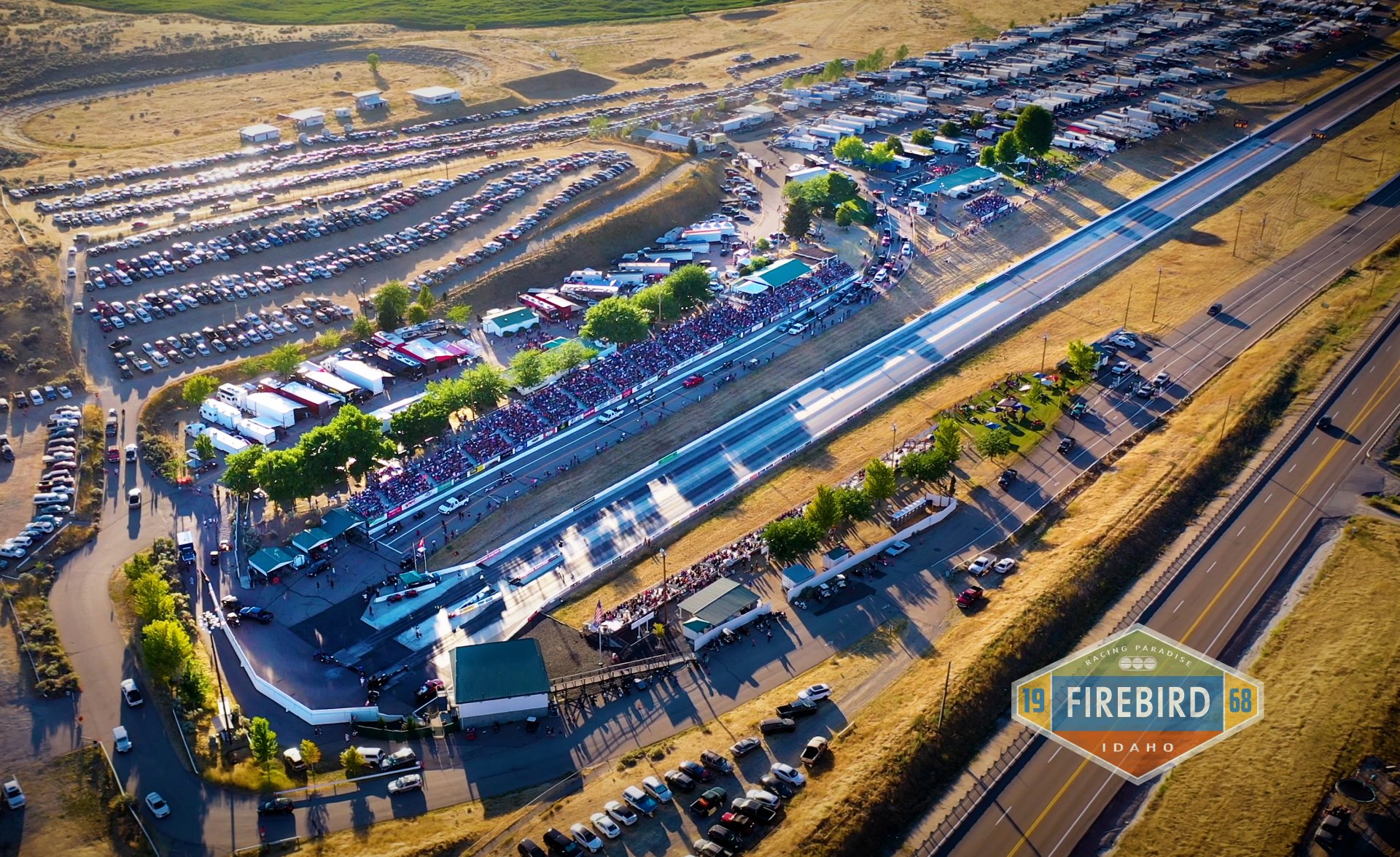The photograph offers a detailed aerial view of an automotive racing complex nestled in what appears to be a rural neighborhood. The focal point is a drag strip that runs diagonally from the bottom left to the top right of the image, bordered by spectator stands on either side. Surrounding the racing area are numerous cars and large trailers, likely belonging to various racing teams. The lot is bustling with vehicles, while the upper right corner features a cluster of truck trailers parked in neat rows. This area seems isolated, with a mix of dirt patches and hills, giving it a somewhat rustic backdrop. Two highways intersect the landscape, with the modern one cutting through prominently and an older, dilapidated one trailing off to the right. As the light of day begins to fade, adding a soft glow to the scene, an emblem located in the lower right corner stands out. It reads "1968 Firebird, Idaho Racing Paradise" and is adorned with blue, red, yellow, and green accents, hinting at the area's rich racing heritage.